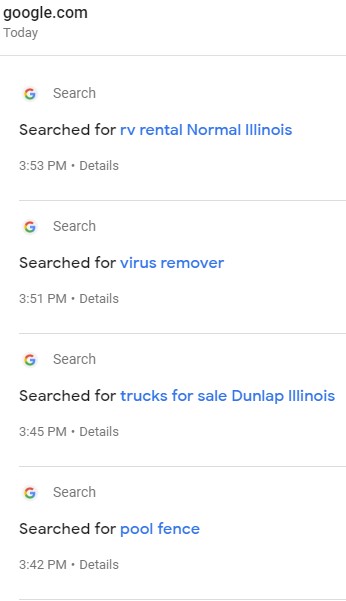A vertical screenshot of an unknown search website displays several recent searches. At the top, the text "google.com" is prominently featured in black letters. Below, the screen captures a series of search entries with the following details:

1. "Search for RV rental, Normal, Illinois, 3:53 PM" 
2. "Search for virus remover, 3:51 PM"
3. "Search for trucks for sale, Dunlap, Illinois, 3:45 PM"
4. "Search for pool fence, 3:42 PM" 

The image is purely textual and lacks any photographic elements, people, animals, birds, buildings, bridges, mountains, flags, banners, signs, billboards, automobiles, motorcycles, bicycles, or airplanes. Its tall, narrow format underscores the list of time-stamped queries.